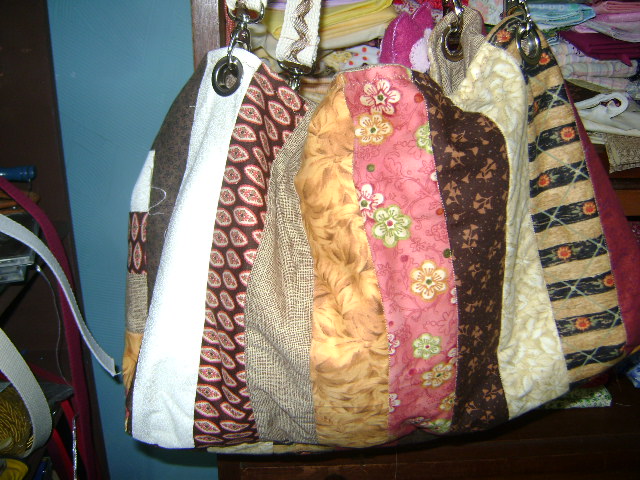The photograph captures a detailed and colorful scene centered around a unique, large handbag that hangs prominently against a blue wall. To the left of the blue wall is a door, and below it, some straps rest atop a stand partially visible in the corner. The central focus is a wooden chair, draped with several bags and perhaps a blanket. One particularly detailed bag features a patchwork of vertically aligned strips, each showcasing distinct colors and patterns.

The vividly designed handbag showcases an array of vertical stripes featuring a variety of intricate patterns: a pure white stripe, a red and brown diamond-shaped floral stripe, a crisscross pattern in white and light brown, yellow autumn leaves, light green and pink-edged flowers on a pink background, white twigs on brown, white flowers on a faded brown and white background, and a final stripe with alternating horizontal rows of brown and blue, each adorned with an orange flower.

The handbag, appearing soft and floppy with an artisanal design, hangs with chrome rings attaching its white straps. The flash from the camera illuminates the center of the image brightly, making the bag's detailed patchwork stand out against the darker, shadowy edges of the photograph. The chair serving as the backdrop adds a rustic touch to the vibrant and eclectic look of the handbag, with the additional bags and blankets enriching the scene with a sense of complexity and depth.